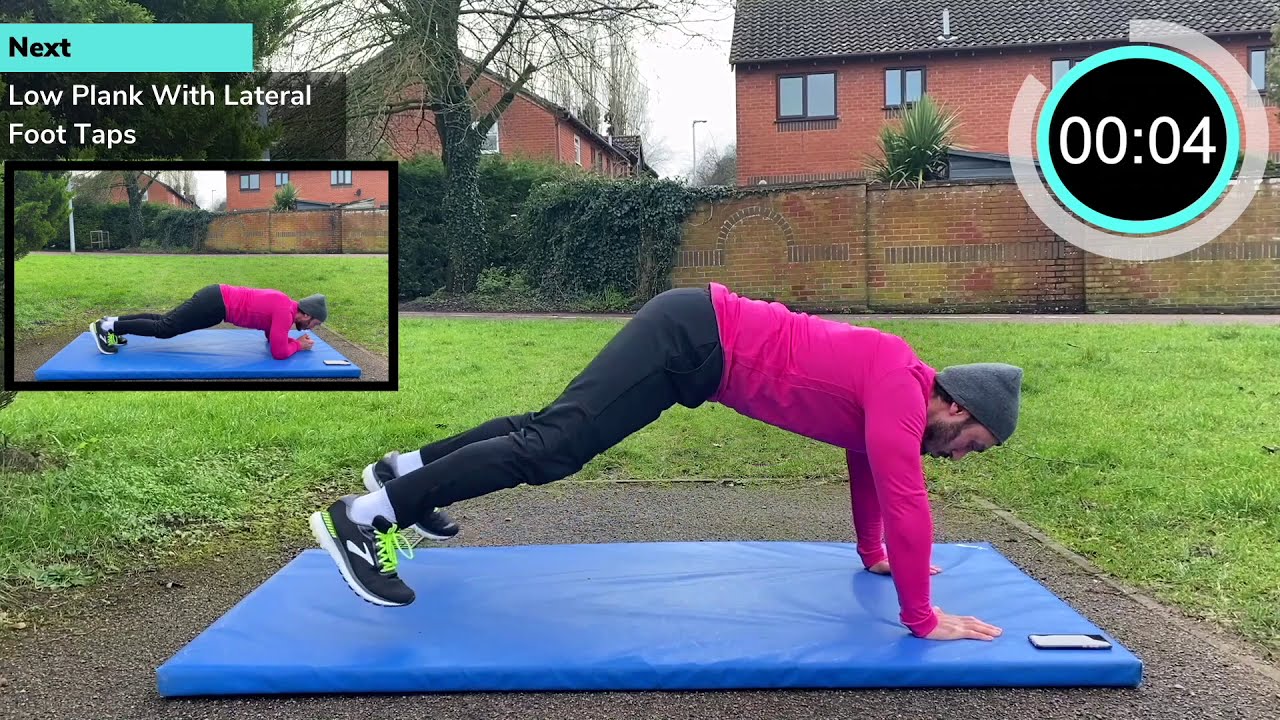The image captures a man engaged in a yoga exercise in his yard, demonstrating a plank position. He wears a pink hoodie, a gray beanie, black pants, and black shoes with green laces, and supports himself on a blue pillowed mat situated in a patchy area blending dirt and grass. A brick wall, heavily adorned with parasitic vines, forms the backdrop, with a barren tree interwoven with the same vines adding to the scene's sparse vegetation. In the top left corner, an inset image previews the next exercise, labeled in a teal banner as "Next: Low plank with lateral foot taps." Concurrently, the top right corner displays a timer reading "0:00:04," enclosed within a circle partially diminished to indicate the passing seconds. Despite the undefined current exercise, the composition effectively conveys a sense of guided fitness in a natural, albeit unkempt, setting.